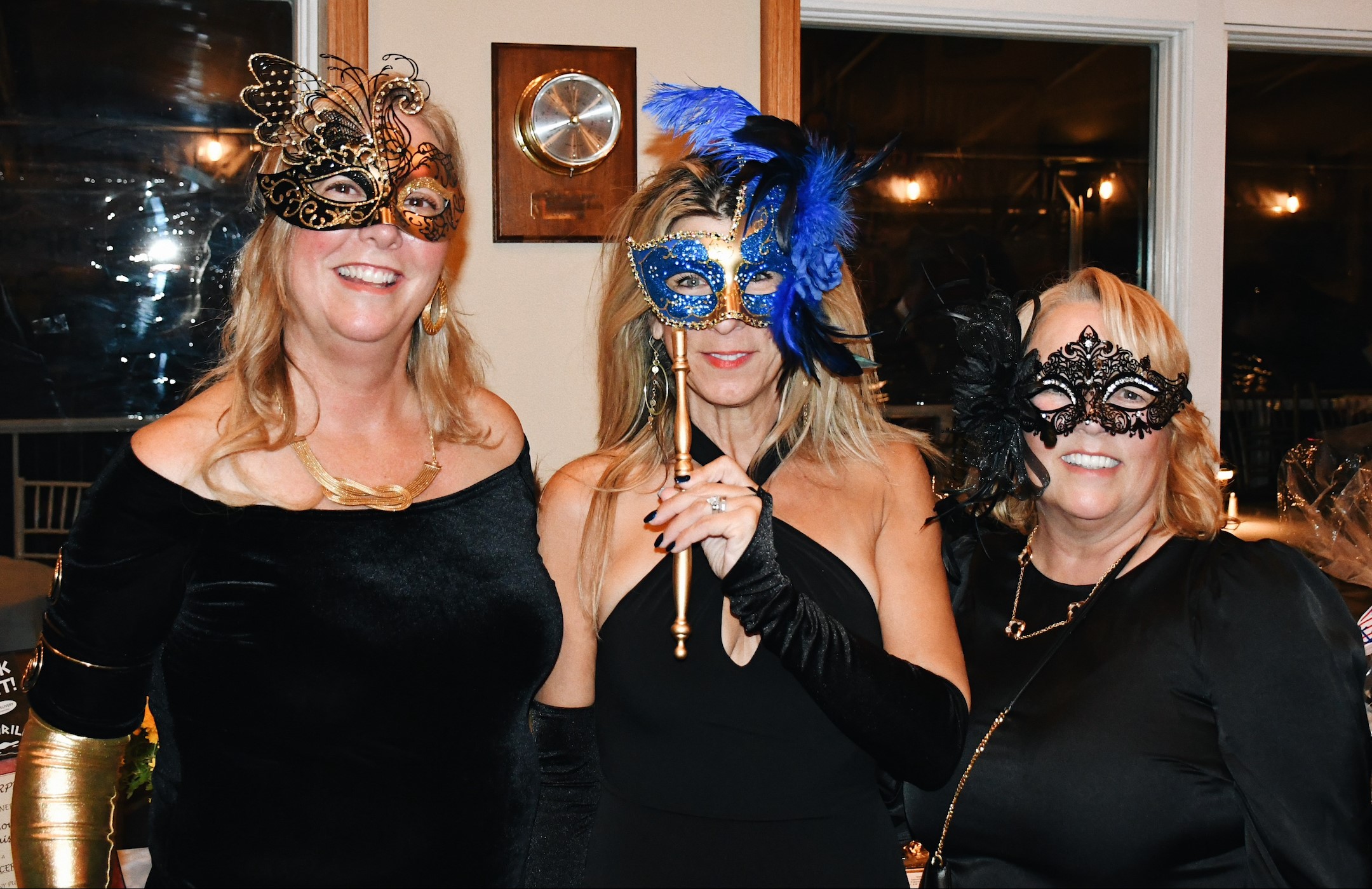The indoor evening photograph captures a masquerade party scene set against a beige wall with floor-to-ceiling windows on both sides, through which outdoor lights indicate it is nighttime. In the center of the image, three blonde women of different heights all don black dresses and distinctive masks. On the left, the tallest woman wears a velvet black dress featuring golden sleeves, paired with a black and gold swan-like mask. The middle woman, dressed in a halter-top black dress and black arm warmers, holds a striking blue and gold mask with a handle, adorned with feathers. The shortest woman on the right sports a long-sleeve black dress and a delicate black lace mask. Each element of their attire and the sophisticated ballroom setting contributes to the festive, enigmatic atmosphere of the masquerade party.